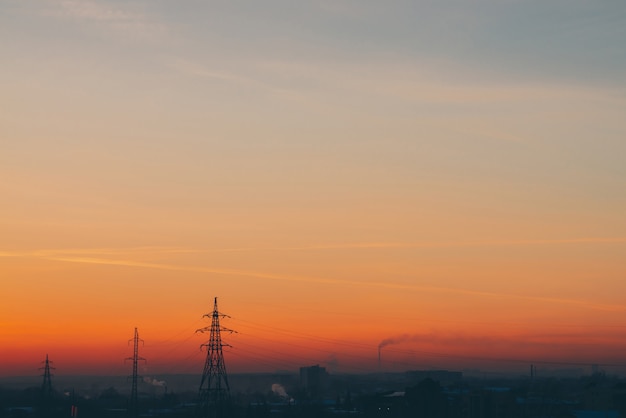The image captures a mesmerizing sunset over an industrial landscape, characterized by a distinctive layered sky and tall electrical towers. At the bottom of the image, the scene is enveloped in darkness, interspersed with at least three prominent electrical towers, some with intricate wire connections at various levels. The foremost tower features a triangular design, while others, including light towers and a narrower structure, stand in the background. Adjacent to these towers, a smokestack releases a plume of smoke, adding to the industrial ambiance. The sky is a captivating gradient, beginning with dark red near the horizon, transitioning to orange, streaked with white and yellow, and finally blending into a soft sea foam green, then teal, and a light greenish-blue at the top. This tranquil yet industrialized scene is punctuated by delicate hues, making it a visually layered capture of a sunset.